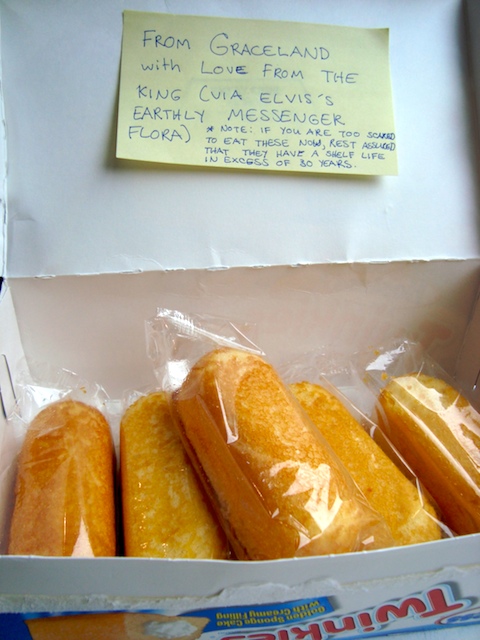The image showcases an opened box of Twinkies displayed upside down, revealing its contents. Inside, five Twinkies are positioned vertically, with four stacked at the bottom and one placed in between. A prominently positioned yellow sticky note is stuck to the inside lid of the box. Written in blue ink, the note reads, "From Graceland, with love from the King, via Elvis's Earthly Messenger Flora. Note, if you are too scared to eat these now, rest assured that they have a shelf life in excess of 30 years," with an asterisk next to the word "Note." The Twinkie packaging features an image of a Twinkie with a visible bite, showcasing its creamy filling, and the word "Twinkie" appears upside down.